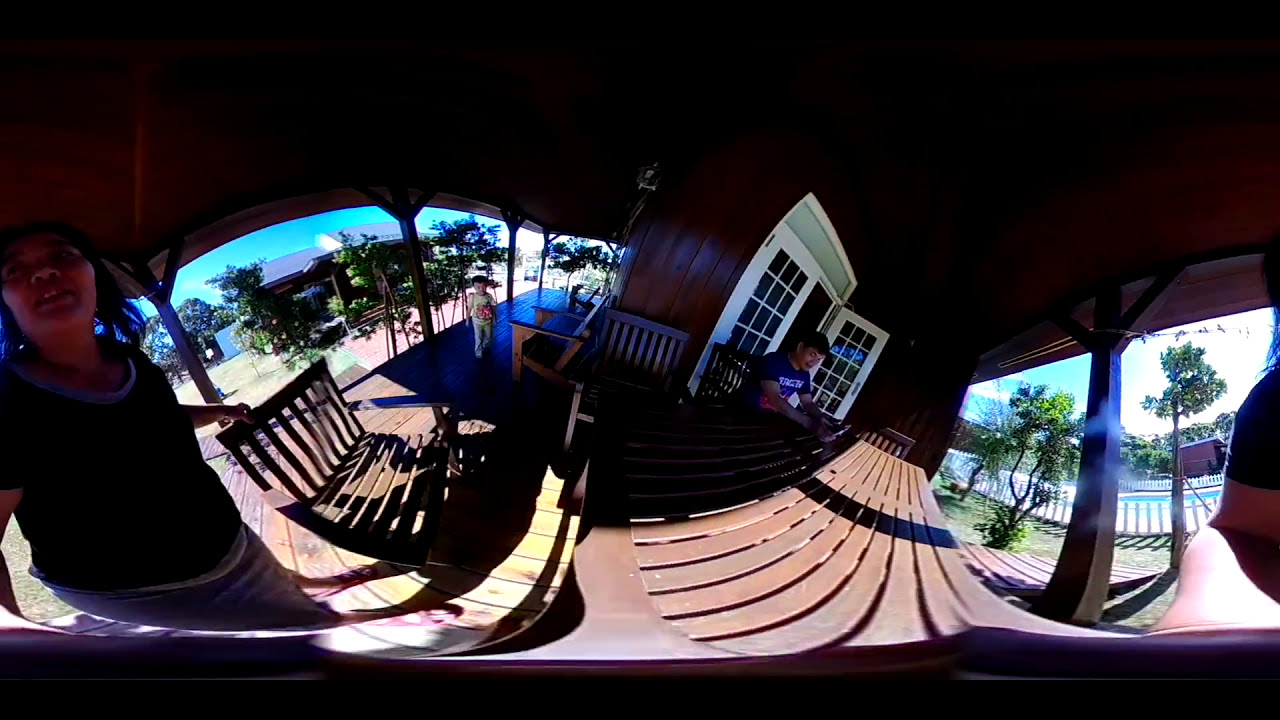This horizontally aligned, wide-angle image captures an outdoor deck or patio area bathed in natural light. Underneath a covered section with a dark brown ceiling supported by metal poles, three people are visible. In the foreground to the left stands a woman with shoulder-length black hair, donned in a black and white short-sleeve top. Her hand rests on a wooden chair, and her mouth is slightly open as she looks upwards. In the middle, sitting at a dark brown picnic-style table made of horizontal wooden slats, an older man with short black hair is engrossed in his phone, which he's holding on the table. He’s wearing a blue t-shirt adorned with white print. To the far right and slightly towards the back, a young child in a yellow and red shirt paired with grey pants walks towards the camera. The background reveals a clear blue sky, several trees to the left, another building that looks like a house or small store, and a set of steps leading up to it. On the far right, beyond the covered area, a pool and fence are also slightly visible.